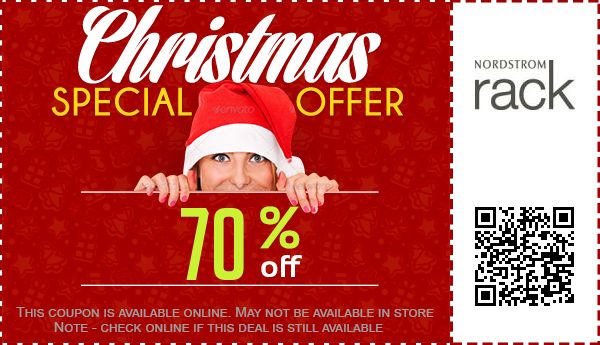The image features a coupon likely printed from a website. The background is a deep red hue with a pattern of dashed black lines. At the top center, "Christmas" is elegantly written in cursive white font. Below this, the text "Special Offer" appears in vibrant yellow. Between the words "Special Offer" is an image of a Caucasian woman with deep blue eyes peeking over an edge. She is wearing a red and white Santa Claus hat and has red-painted nails. Beneath this, the text "70%" is displayed in the same yellow color, followed by "OFF" in white.

At the bottom, in gray text, it states, "This coupon is available online. May not be available in-store. Check online if this deal is still available." On the right-hand side of the coupon, there is a white area featuring the Nordstrom Rack logo. Adjacent to the logo is a QR code intended to be scanned with a smartphone to access further details or the offer online.